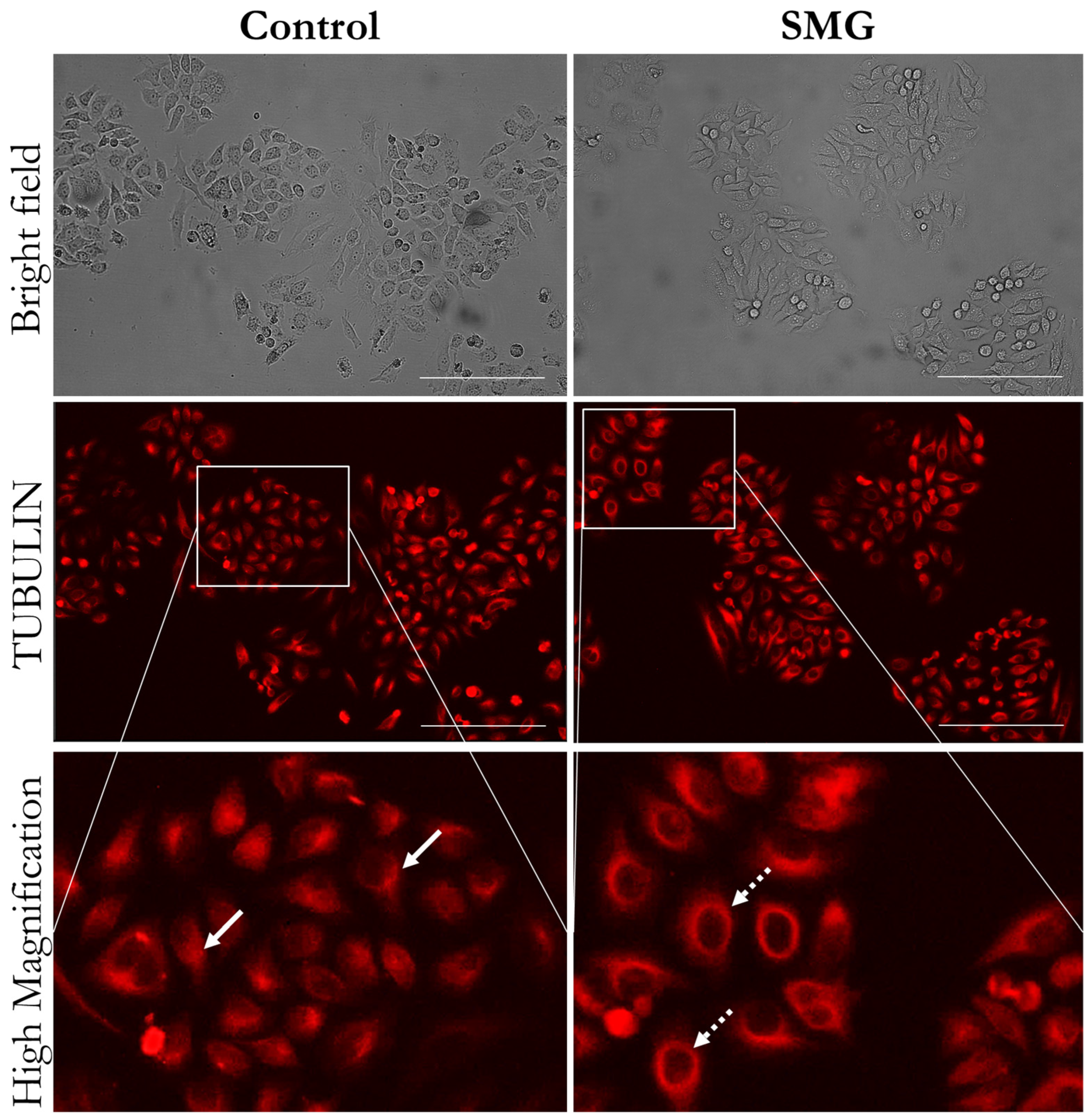This image appears to be a scientific diagram, potentially related to blood cells, organized in a 2x3 grid layout. The left column is labeled as 'Control' and the right column as 'SMG.' Each column is divided into three rows corresponding to different imaging techniques and magnifications. The top row is labeled 'Bright Field,' showing a grayscale microscopic view with distinguishable patterns, possibly of cells. The middle row is labeled 'Tubulin,' and it displays structures highlighted in red, likely indicating tubulin proteins within the cells. The bottom row is 'High Magnification,' providing a closer and more detailed look at cellular structures, highlighting areas where components like oxygen and tubulin might be present. The comparison between 'Control' and 'SMG' across these different imaging types suggests a focus on identifying differences in cellular structures and composition.